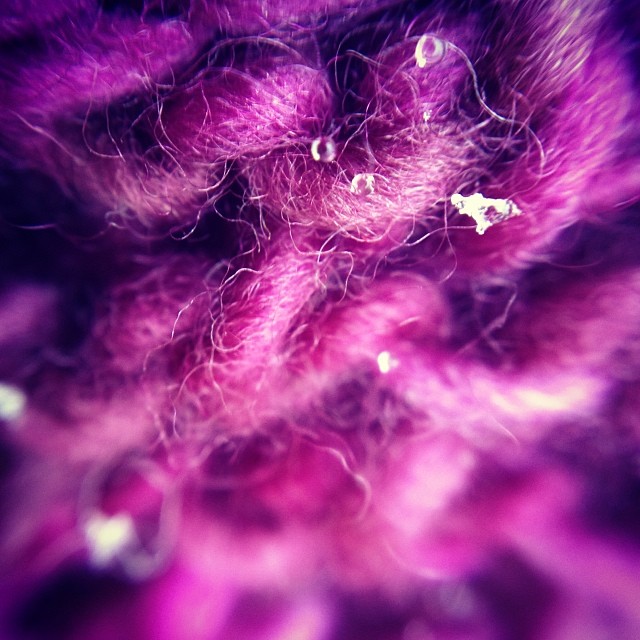This image showcases a highly magnified close-up of what appears to be purple yarn or carpeting, woven intricately with visible fibers protruding like fine, hair-like strands. The fabric's texture is detailed, showing the interwoven pattern reminiscent of a chain-link fence, with threads passing over and under each other. Towards the upper part of the image, there are three noticeable water droplets resting on the fibers, adding a reflective quality. Additionally, small splotches of white, possibly ice or additional water droplets, are scattered, particularly in the upper right section. The color palette of the yarn varies from light purple to very dark purple, almost black in some densely packed areas. The image becomes increasingly blurry at the edges, emphasizing the sharp, detailed focus in the center. This intricate close-up captures the tiny fibers and the woven structure vividly, illustrating the complex texture of the material.